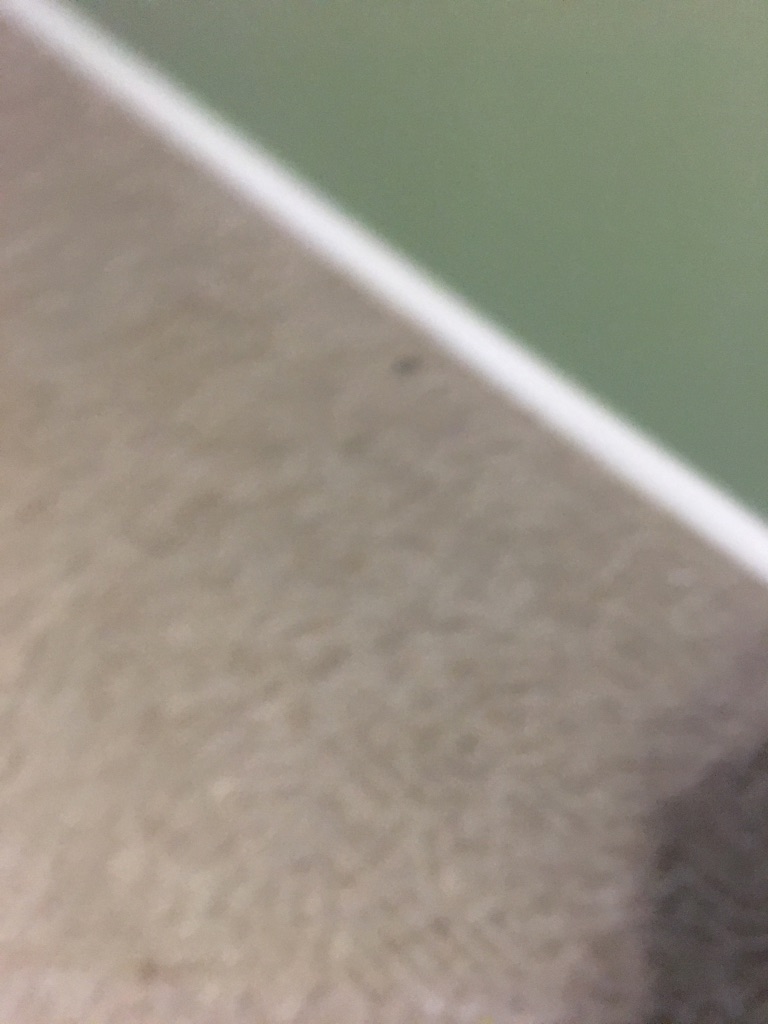This image features a somewhat blurry composition, where the top right-hand corner is dominated by a solid green triangular shape. Adjacent to this shape is a distinct white painted line that traverses across the scene. Below the line is a gray area peppered with darker gray dots, creating a textured effect. The gray gradient intensifies towards the top and lightens progressively as it reaches the bottom of the image. Adding to the complexity, there is a prominent dark black circle located near the white line. To the right of the frame, a shadow encroaches into the scene, adding an element of mystery and depth.